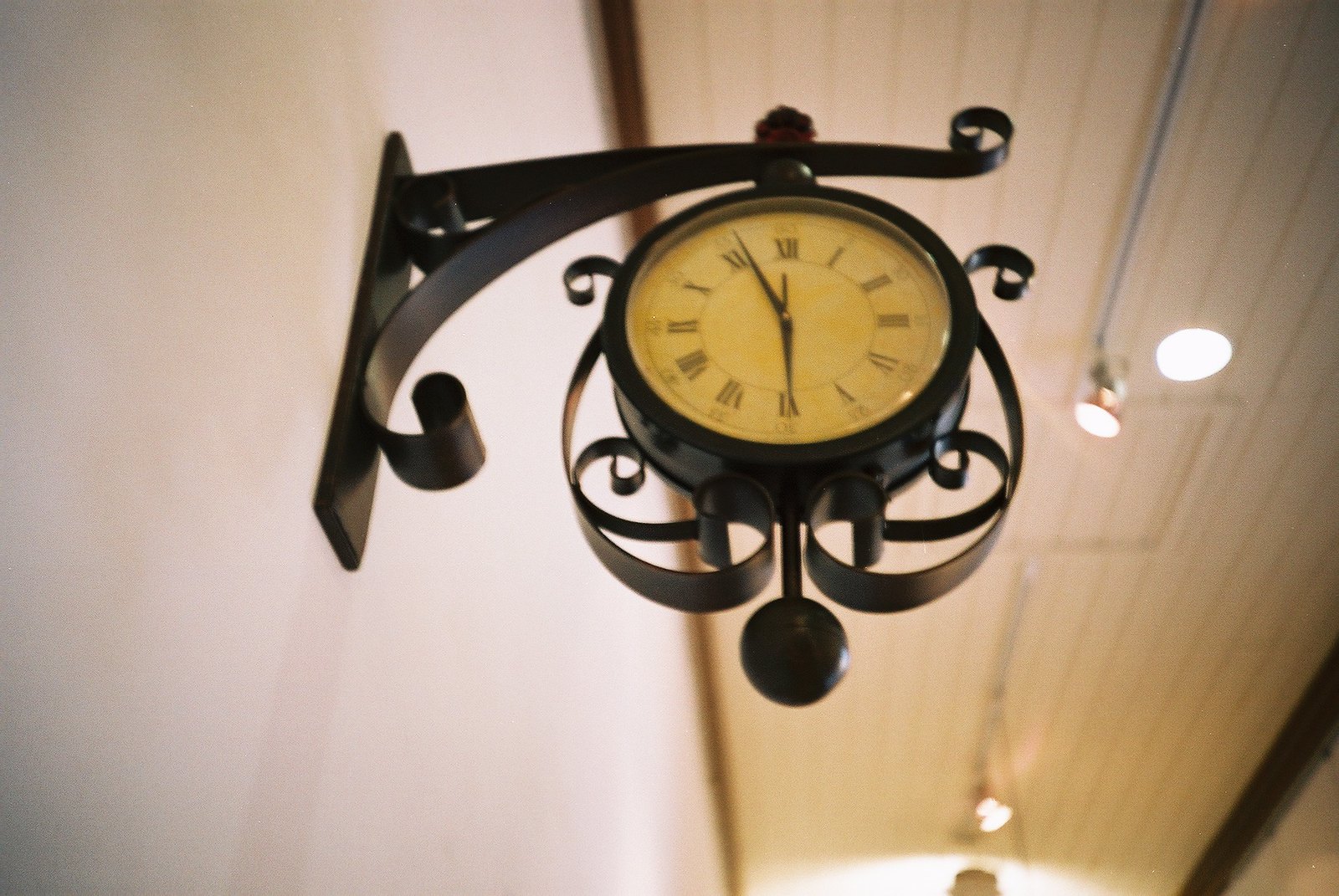The photo depicts a small, round black metal clock with a yellowed face, showcasing Roman numerals for hours. It's mounted on a decorative, swooping metal arm attached to a rectangular base on a white wall. The clock, slightly ornate with metal spirals on its sides and bottom, indicates a time close to 6:52. A black metal ball hangs from the bottom of the clock. Above this indoor scene, there's a wooden ceiling with visible track lighting comprising two lights on the left side. The setting appears to be an indoor area reminiscent of a train station or platform, characterized by additional decorative elements and practical fixtures like round light fixtures and electrical piping. The environment features dark brown trimmings on both the left and right sides.